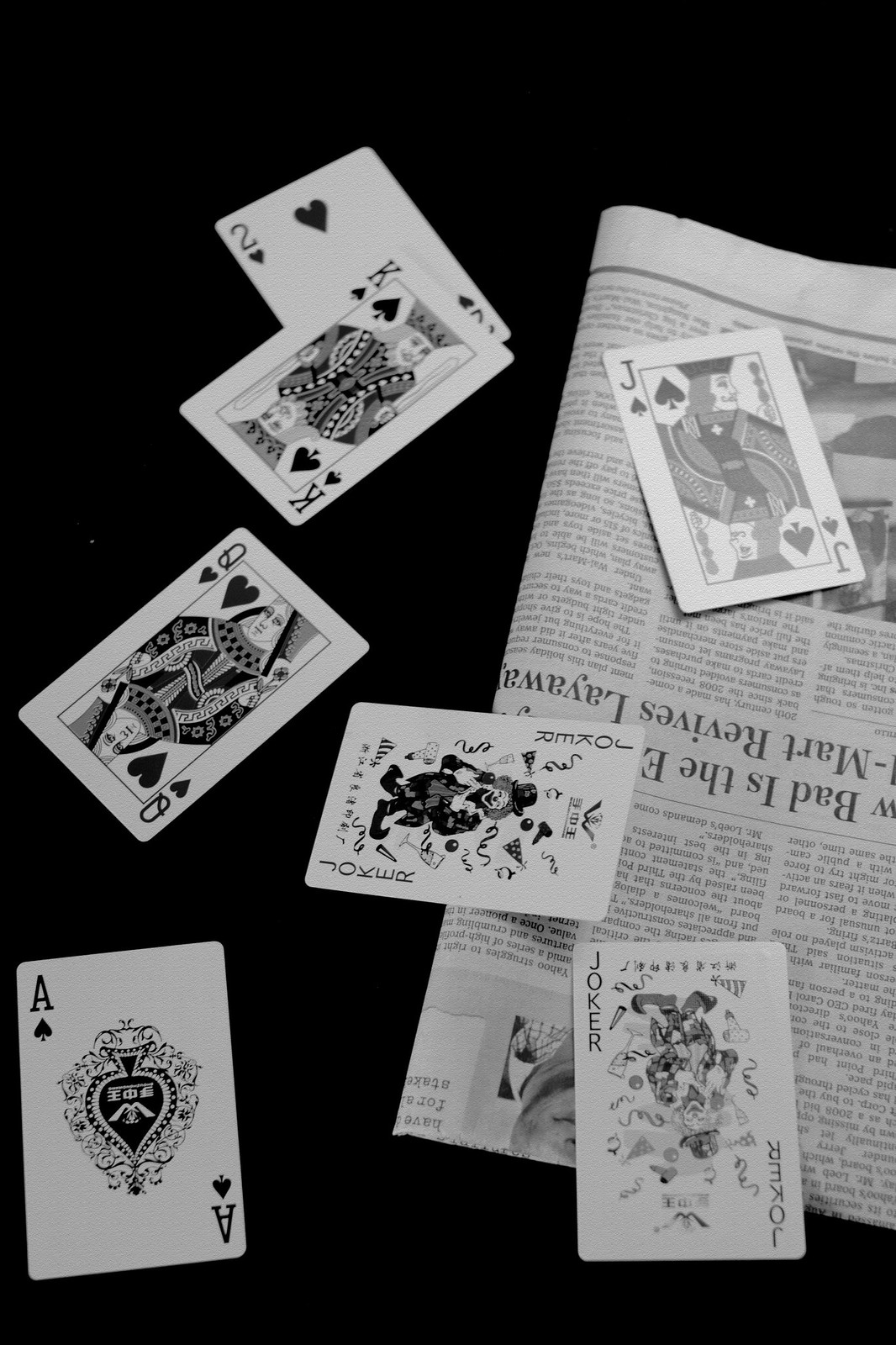In this striking black-and-white photograph, a dark black background envelops the scene, casting a dramatic shadow over what appears to be a table or desk, the exact identity of which remains ambiguous. Scattered haphazardly across the surface are an array of playing cards, displaying no discernible pattern indicative of a card game. The cards include a two of hearts, a king of spades, a jack of spades, a queen of hearts, an ace of spades, and two joker cards, all seemingly carelessly dispersed. Peeking from beneath the jack of spades and the two joker cards is a partially visible newspaper. Snippets of text from two articles can be deciphered, with one focusing on the economic challenges faced by Walmart, compelling the retail giant to revive its layaway program, evidenced by the partial headline: "How bad is the economy? Walmart revives layaway." The top fragment addresses an individual named Mr. Loeb and his pressing demands, although the exact details remain obscured. This thoughtfully composed image blends elements of randomness and intent, showcasing the interplay between everyday items like playing cards and newspaper clippings, captured timelessly in monochrome.